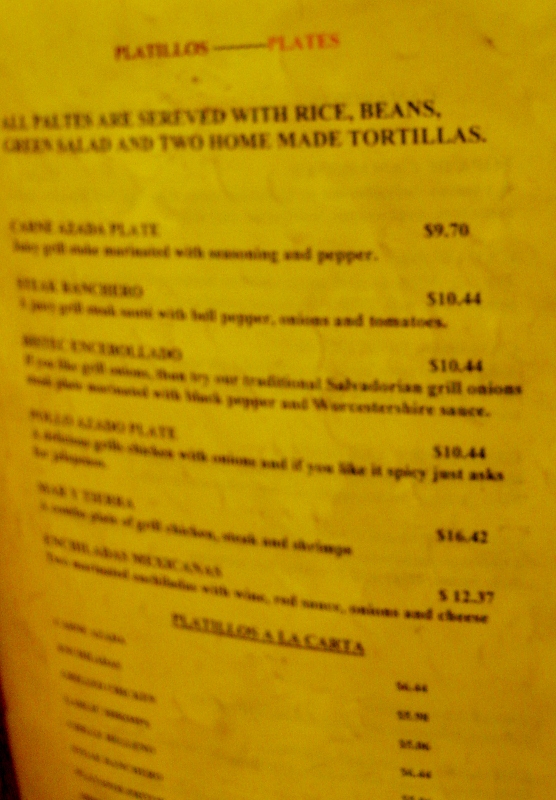This photograph captures a blurry close-up of a yellowish-orange menu, likely distorted by improper white balance settings during the photo-taking process. The menu surface appears worn, exhibiting slightly dark grey lines resembling pencil marks. At the top of the menu, the word "Plateaus" is in red, followed by a black line, and then the word "Plates" in orange. Beneath these headings, the text reads: "are served with rice, beans, green salad, and two homemade tortillas," although it is largely illegible due to the blurriness.

The menu items include:
1. "Carne Asada Plate" priced at $9.70, with the description being illegible.
2. Something "Ranchero" priced at $10.44, ending with "peppers, onions, and tomatoes."
3. An unreadable item, also priced at $10.44.
4. Another illegible item referred to as a plate with a description noting, "If you like it spicy, just ask for jalapenos," priced at $10.44.
5. Another unreadable item priced at $16.42.
6. An item partially readable as something "Mexicanos," priced at $12.37.
   
Beneath these plates, the menu lists "Plateaus a la Carta" with items that are too blurred to discern.